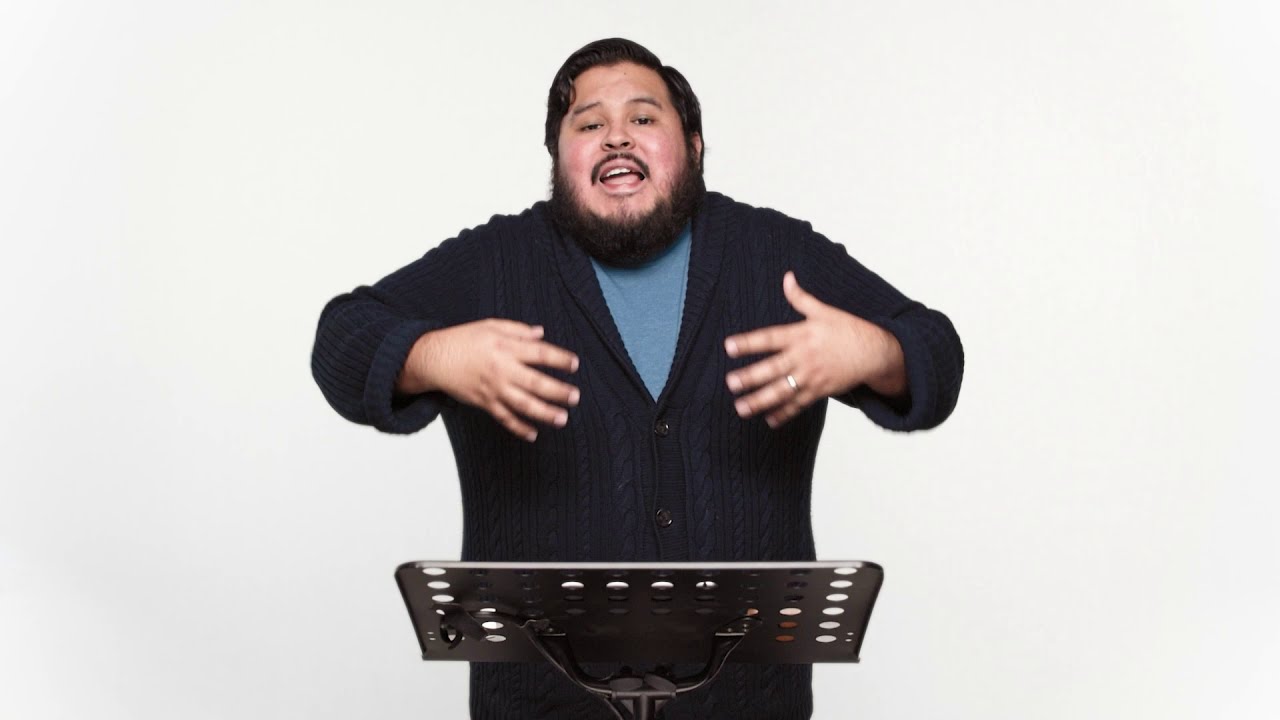In the image, a man stands behind a perforated metallic podium, visible from the torso up. He appears to be of Hispanic or Indian descent, with dark hair, a mustache, and a beard. His face shows an exasperated, excited expression as he speaks or sings, with his mouth open, revealing his top row of teeth and tongue. His head is slightly tilted back. He is dressed in a dark blue, button-up, V-neck cardigan sweater over a lighter blue shirt. A gold wedding ring adorns the ring finger of his left hand. His elbows are bent with his hands at chest level, gesturing expressively. The light blue background contrasts with his figure, emphasizing his presence at the podium.